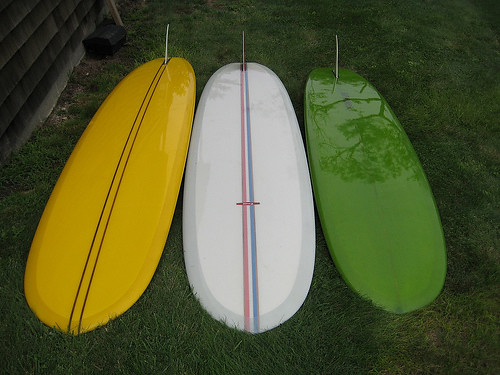In this image, we see three vibrant surfboards laid out vertically next to each other on a well-kept grassy area, adjacent to a fence and a wooden house wall. The grass is lush and green, providing a stark, natural contrast to the colorful surfboards. From left to right, the first surfboard is bright yellow with two thin black stripes running down the middle, though the fin color is challenging to distinguish, possibly white. The middle surfboard is white, featuring thicker central stripes of red and blue. The third surfboard on the right is a bright green, more vivid than the grass, with a subtle reflection of a tree and its branches visible on its surface. The surfboards dominate the relatively dark image, with all colors prominently standing out amidst the green grass. Additionally, to the left of the surfboards is a wooden house wall with dark brown, faded panels and a gray cement base. A black object, potentially a toolbox, is visible just above the surfboards.